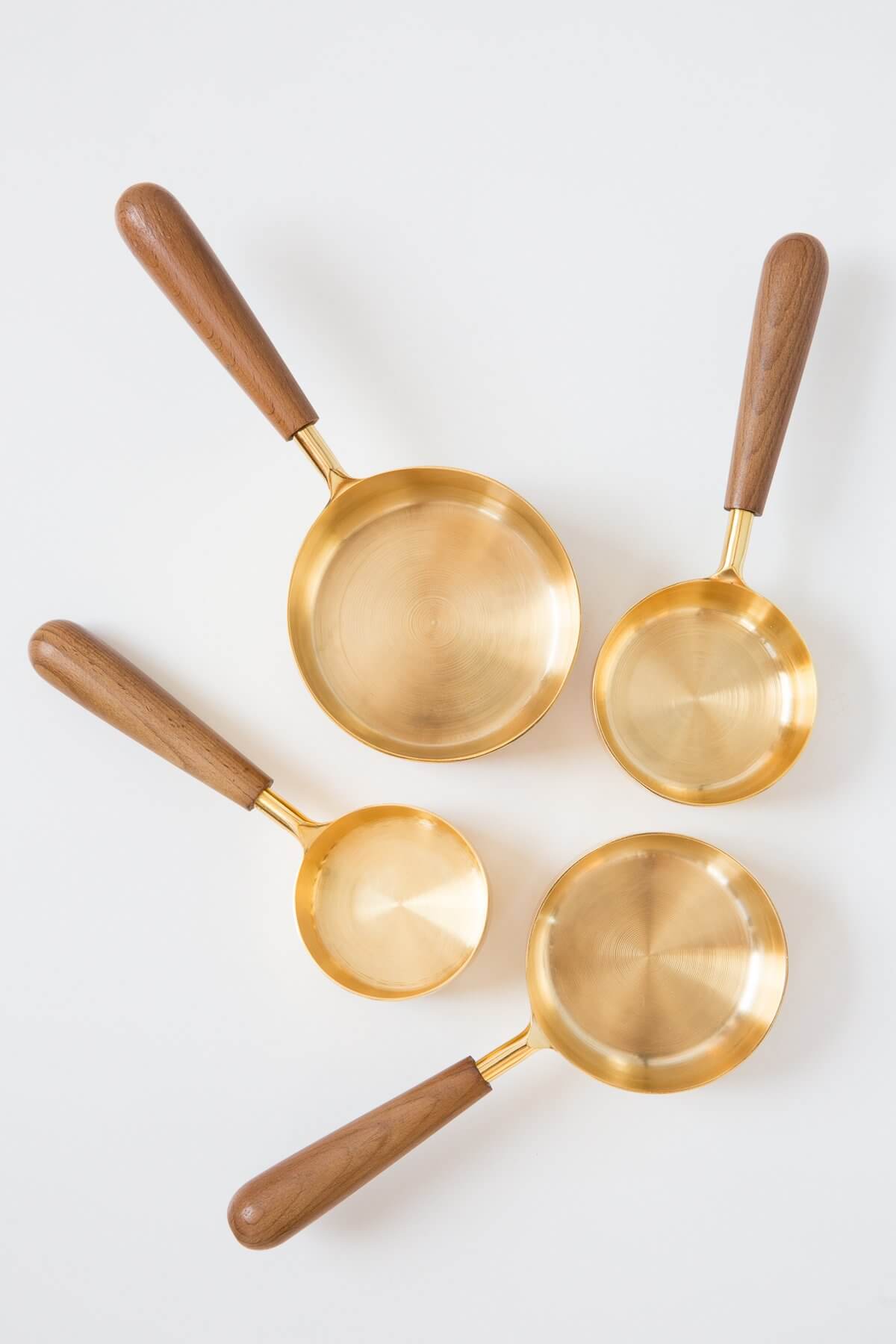The image features four golden frying pans or skillets, each varying in size from very small to large. These shiny and new pans are placed on an off-white surface, arranged in a way where each wooden handle, displaying a distinct wood grain and about the same length irrespective of the pan's size, points in a different direction. The top left pan's handle directs toward the top left corner, while the handle of the bottom left pan angles upward but inward, towards the center. The top right pan's handle points toward the top right corner, and the bottom right pan's handle extends toward the bottom left corner. The golden pans glisten against the surface, casting shadows to the right, and their round smooth wooden handles contribute to an elegant finish, giving the array a polished, cohesive appearance.